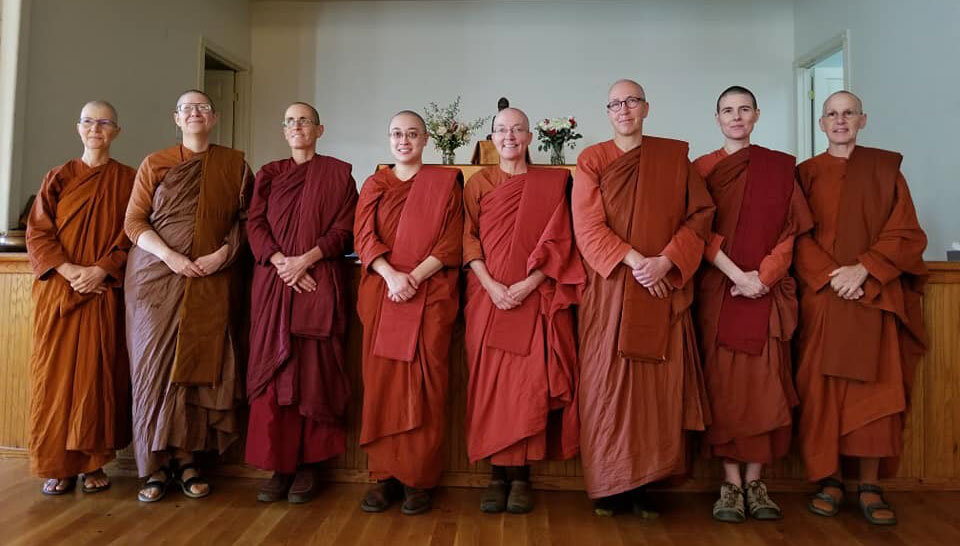This landscape photograph captures eight individuals who appear to be Buddhist monks standing on a wooden floor. The group comprises both males and females, identifiable by their closely shaved heads, some completely bald, while others have very short hair. All are Caucasian and garbed in traditional red and reddish-brown robes that extend almost to their feet. Some of the group members wear glasses, and their footwear varies between sneakers and sandals.

The monks are arranged in a row, looking straight into the camera, with their hands crossed over their waists. Behind them is a wooden structure that reaches about waist height, possibly serving as a desk or a stage, blending into an interior space characterized by white walls. In the background, there are two doorways and a few vases with flowers, contributing to the serene and simple ambiance of the room.